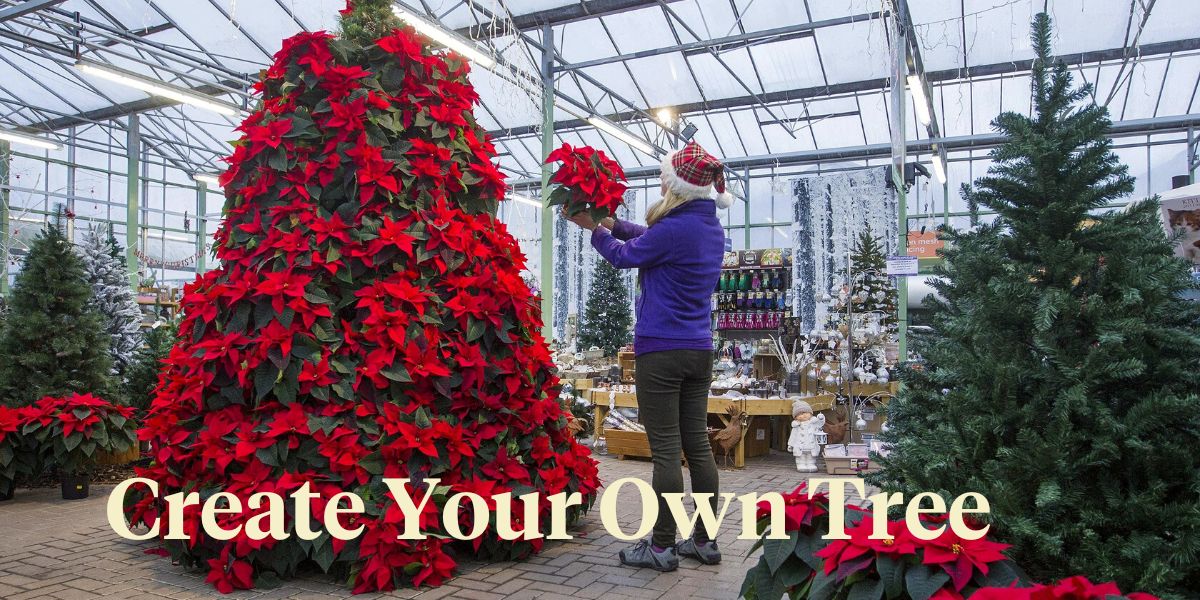The photograph captures the interior of a grand glass-walled building, resembling a greenhouse but clearly not one. The space is densely decorated with various Christmas trees, each adorned with festive red ribbons and some forming unique shapes. Central to the image is a colossal Christmas tree entirely made of poinsettias. Below this striking tree, large white letters spell out "Create Your Own Tree." 

A woman stands in the foreground, facing the poinsettia tree, dressed in a purple long-sleeve jacket, dark brown pants, light blue sneakers, and a plaid Santa hat. She holds a poinsettia plant, seemingly poised to add it to the intricate poinsettia tree, her blonde hair peeking out from under her hat. The ground beneath her feet is paved with small red bricks.

To her right stands a traditional Christmas tree, with poinsettias at its base, and to her left, in the background, other decorated Christmas trees can be seen. The far wall is adorned with garlands, ornaments, and various decorations, evoking a festive atmosphere. A table behind the woman is laden with decorations, likely for purchase, suggesting that this space is designed to inspire and assist visitors in creating their own holiday tree masterpieces.